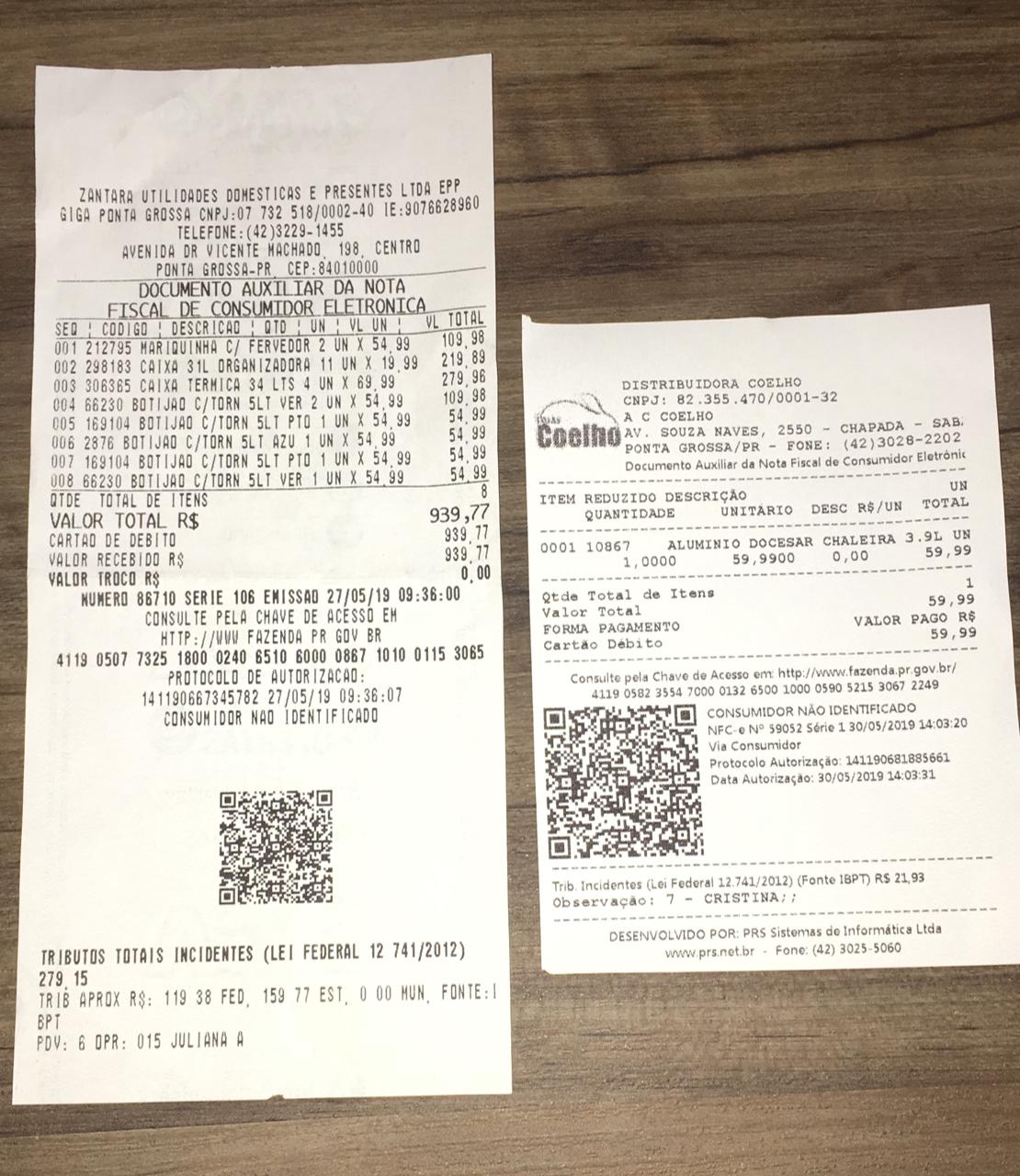This image features two receipts laid out on a brown wooden table, with both receipts written in a foreign language, possibly Spanish. The receipt on the left is longer, displaying a detailed itemized list along with the total amount of $939.77 in a currency that could be pesos. Towards the bottom of this longer receipt, there's a QR code followed by some additional text. The shorter receipt on the right lists a single item priced at $59.99 and also features a QR code toward the bottom. Above the store name on this shorter receipt, there's a logo that appears to read "COELHO." Both receipts include purchase details such as the store's name, address, and phone number at the top. The left receipt's length compared to the right creates a noticeable contrast in their respective heights.